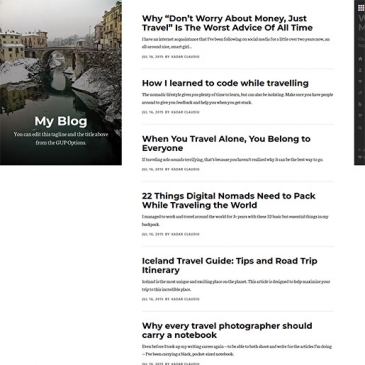In this screenshot, we see an engaging image from a blog interface. In the upper left corner, there's a rectangular photo of an old city bisected by a river flowing vertically through the center, with an ancient bridge spanning the water. Below this evocative image, the words "My Blog" are prominently displayed in white text. To the right of the cover photo, a series of blog titles are listed in bold black text. The titles, running from top to bottom, are as follows: "Why 'Don't Worry About Money, Just Travel' is the Worst Advice of All Time," "How I Learned to Code While Traveling," "When You Travel Alone, You Belong to Everyone," and "22 Things Digital Nomads Need to Pack While Traveling the World."